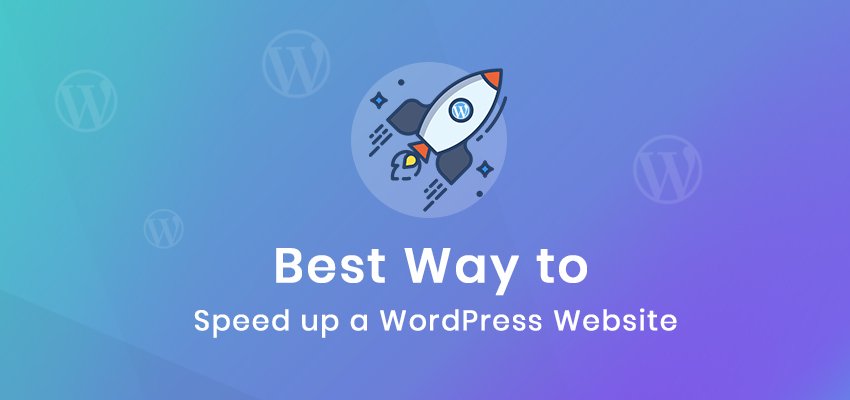This image showcases a visually striking cover icon with a vibrant background featuring an array of colors, including turquoise green, and shades of purple and blue. Prominently displayed are several 'W' characters in various sizes—small, medium, and large—stylized in elegant cursive and each encircled. At the center of the image, a white spaceship with red tips at both the top and bottom captures attention. Overlaid text reads, "Best Way to Speed Up a WordPress Website," providing a clear and direct message. The overall aesthetic is both captivating and informative, combining bold visuals with concise text.